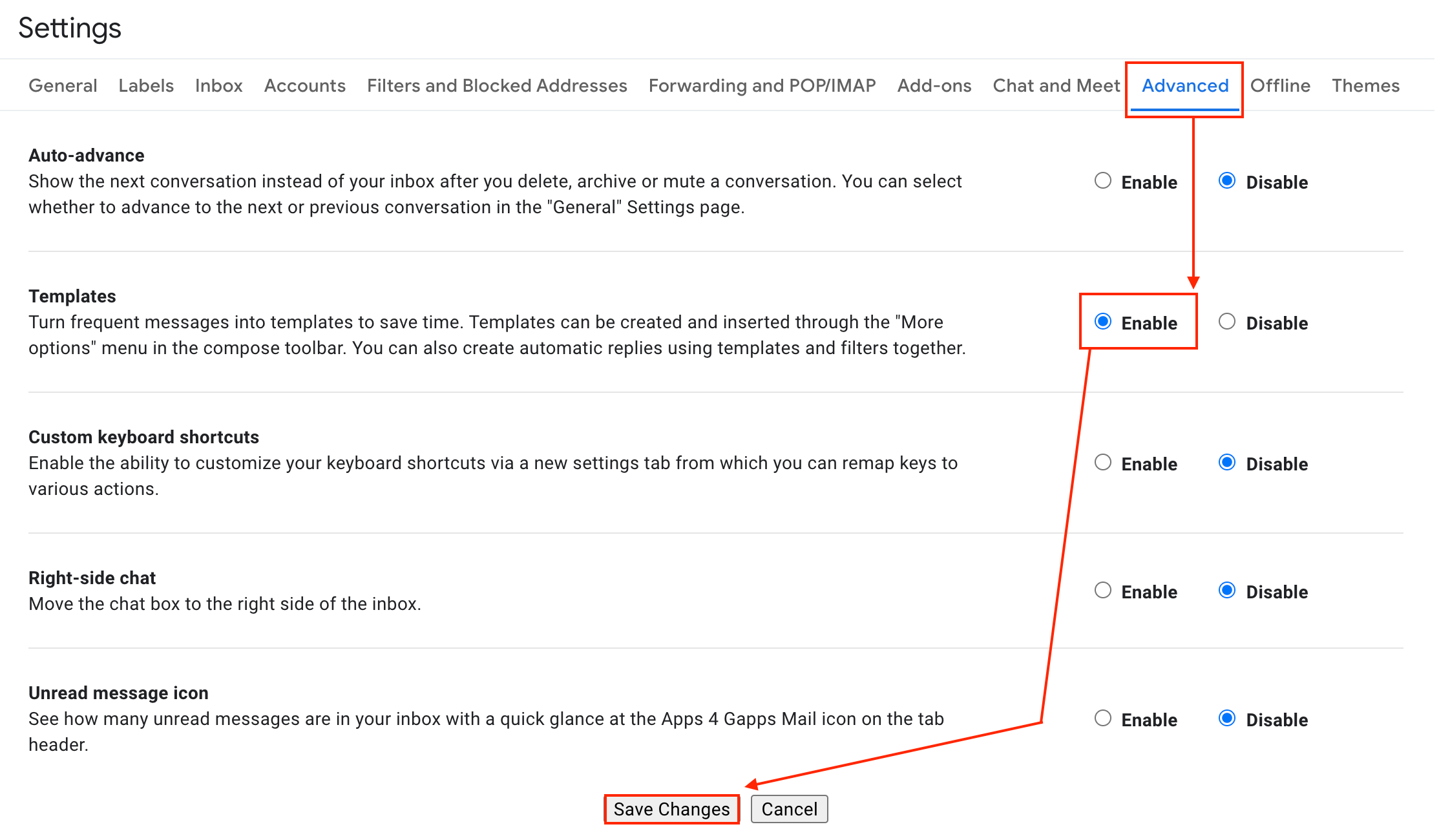This image depicts the settings page of an application, featuring a predominantly white background with primarily black and gray text. The interface is structured with multiple sections, including a menu bar on the left side that lists 11 different categories: General, Labels, Inbox, Accounts, Filters and Blocked Addresses, Forwarding and POP/IMAP, Add-ons, Chat and Meet, Advanced, Offline, and Themes. In the image, the 'Advanced' category is selected, highlighted in blue and underlined, while the other categories are written in gray.

Under the 'Advanced' section, there are five options displayed, accompanied by radio buttons allowing users to toggle between 'Enable' and 'Disable'. These options include: Auto-advance, Templates, Custom Keyboard Shortcuts, Right-side Chat, and Unread Message Icon. Each option name is written in bold black, followed by a short description in a dark gray text.

The current configuration shows that all options are set to 'Disable', except for 'Templates', which is set to 'Enable'. This detailed layout ensures users can easily identify and modify their settings preferences within the 'Advanced' category.